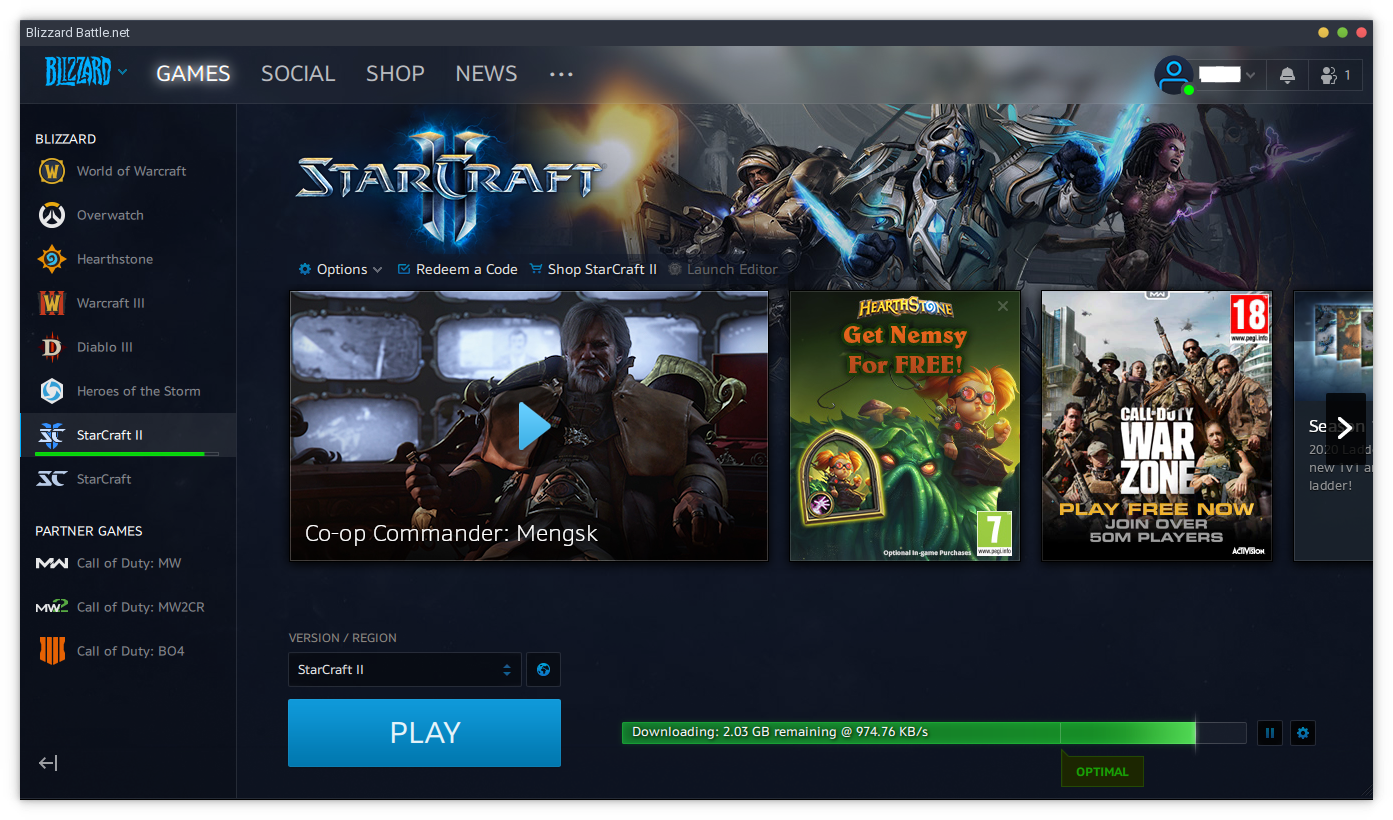The image features a user interface with a grey border at the top. On the top left, the text "BLIZZARD" appears in blue capital letters. To its right, the words "Games," "Social," "Shop," "News," and an ellipsis are displayed in a row. In the top right corner, there are three circles - yellow, green, and red, likely representing status indicators or action buttons.

Along the left column, a list of popular Blizzard games is shown: "World of Warcraft," "Overwatch," "Hearthstone," "Warcraft 3," "Diablo 3," "Heroes of the Storm," "Starcraft 2," "Starcraft," and "Partner Games." Below this, specific Call of Duty game titles are listed: "MW," "MW2CR," and "BO4."

In the center of the interface, a light blue box with white capital letters prominently displays the word "PLAY." Above this button, another box is labeled "Starcraft 2."